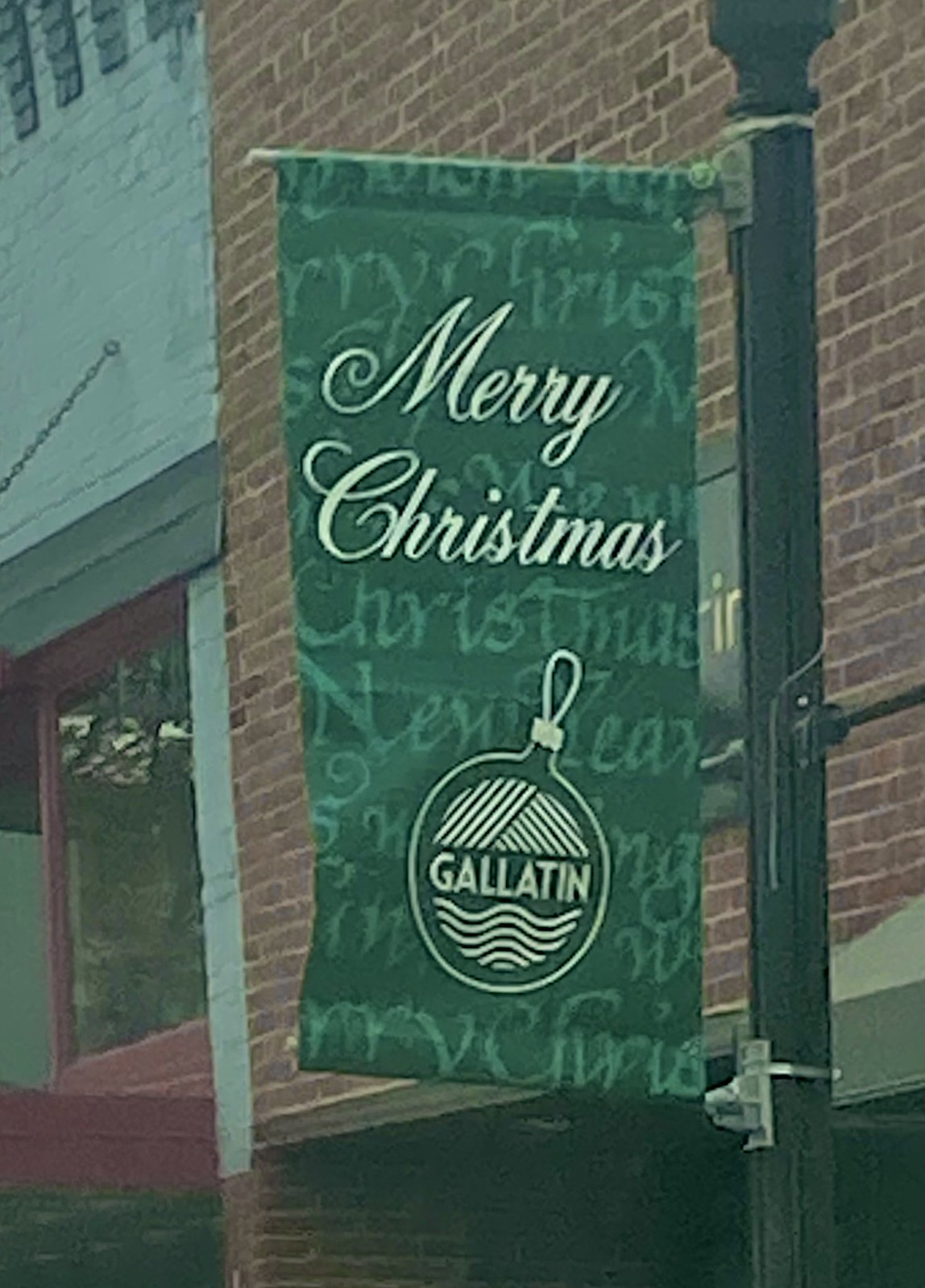The image features a festive green banner hanging from a black streetlight pole, though the light itself is not visible. The banner is affixed to the pole with visible clamps and is supported by an upper and a lower horizontal pole. The banner reads "Merry Christmas" in light-colored letters and features a round Christmas ornament that says "Gallatin." Adjacent to the pole is a red-trimmed window, which is empty. Above this window, a chain extends from the wall but does not connect to any visible item. The scene is set against a tall brick wall, obscuring the store beneath.